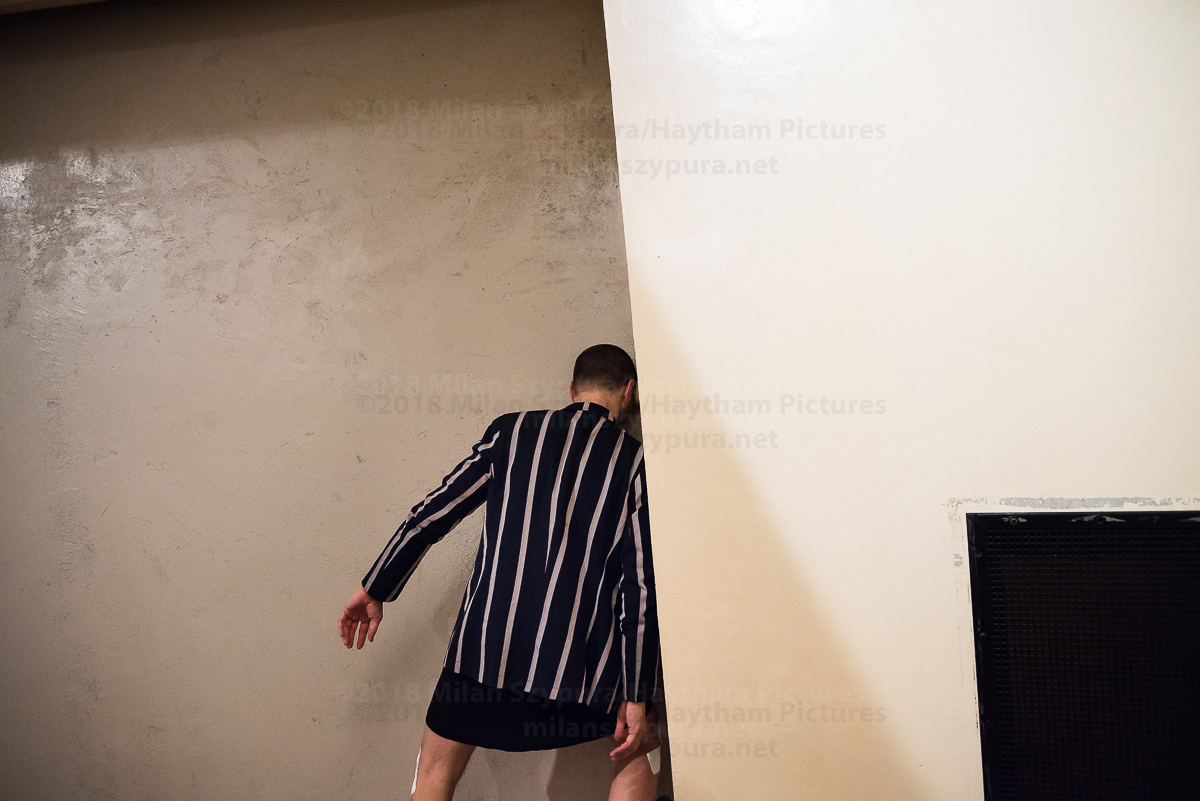The image is a horizontal, slightly angled photograph depicting the back of a man as he interacts with a wall. He is dressed in knee-length shorts and a long-sleeved navy blue dress shirt with white vertical stripes. His black hair and the back of his head are visible as he leans the right side of his body, including his shoulder and head, against a slightly slanted wall. The wall, which displays some wear and tear, is predominantly white on one side and a darker cream color on the other. In the bottom right corner of the image, there is a black section that appears to be part of the wall, possibly resembling drywall. There is text on the wall that reads "Haytham Pictures" in grey, overlapping the scene and adding a sense of mystery to what he might be trying to accomplish in this dimly lit space.